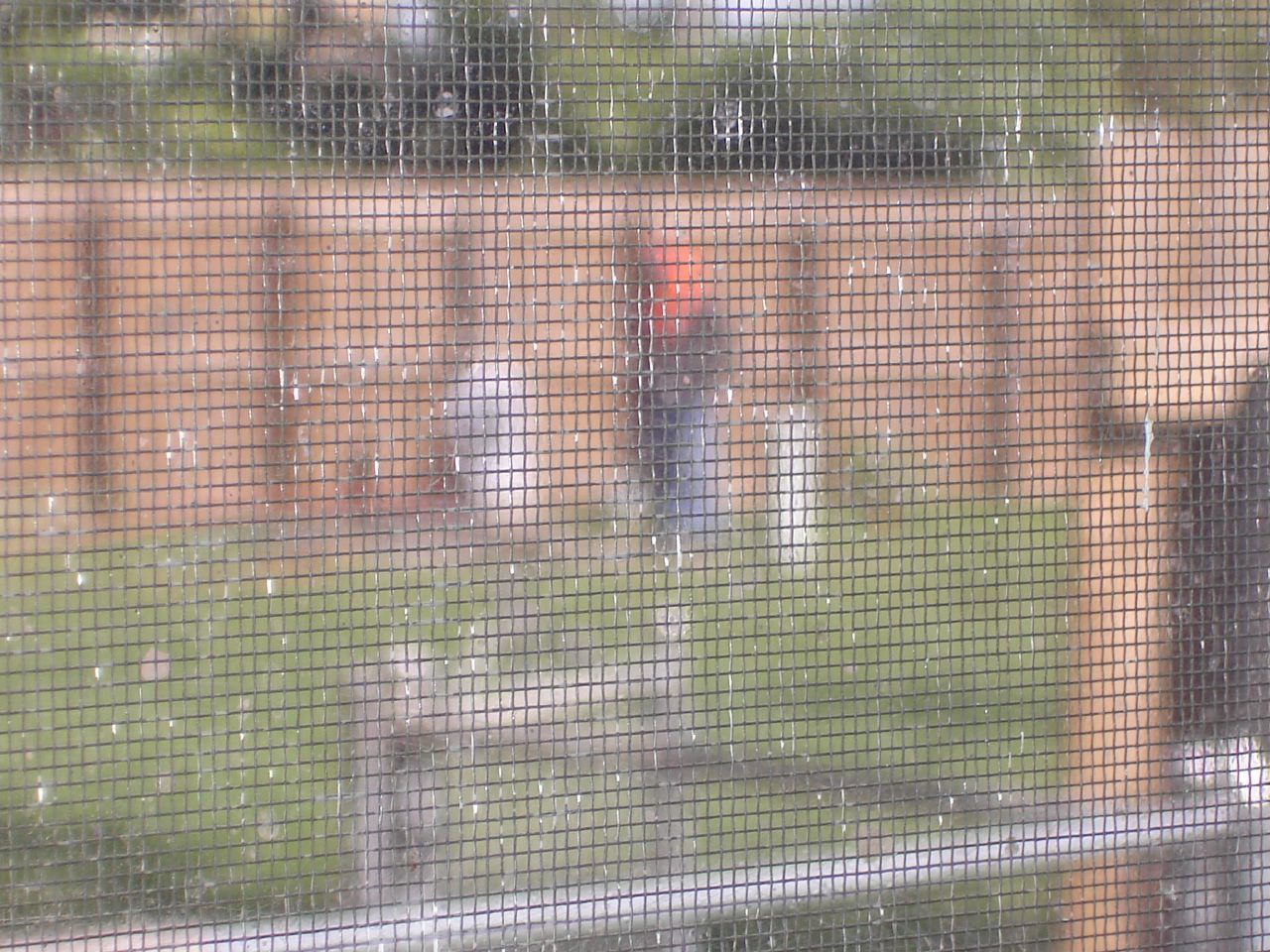This is a blurry image taken through a close-up metal screen or possibly a fiberglass window screen that sharply focuses on the mesh while the background remains out of focus. The screen itself is somewhat dirty and broken, with sections appearing white and the rest a dark gray. Beyond the screen, there is a backyard surrounded by a wooden brown privacy fence, with darker posts visible. In this backyard, a figure, who is difficult to make out clearly, is standing. The person appears to be wearing a black long-sleeve shirt, blue jeans, and has an orange or red object on their head. The ground is covered in green grass with no significant details, and there are several white and brown posts or objects scattered around, some reaching hip level relative to the figure. The tops of trees can be seen in the background above the fence.